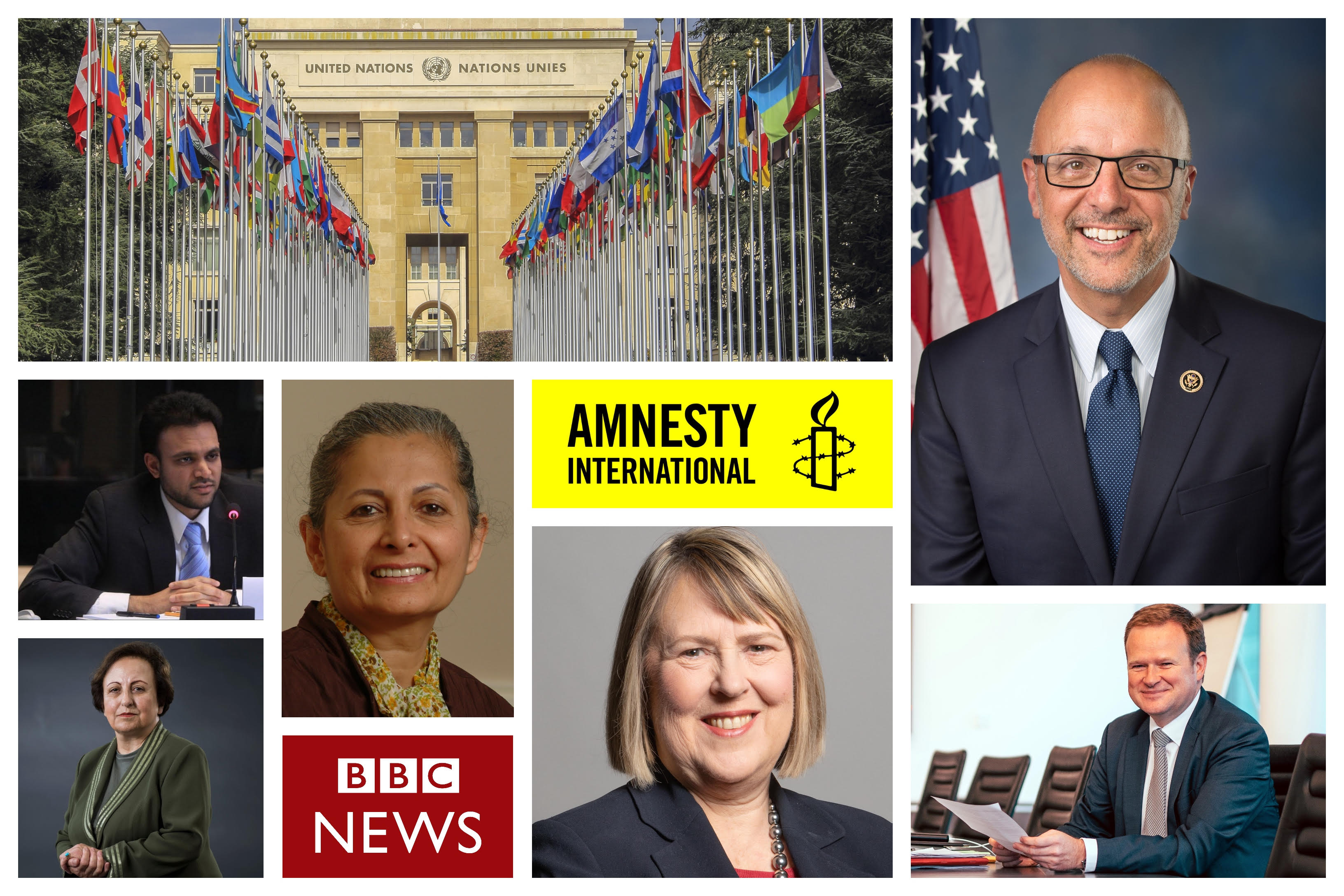The image is a detailed collage consisting of 10 photographs arranged in a grid-like pattern, illustrating various prominent figures and iconic symbols. The central focus is an outdoor photograph of the United Nations building, featuring both sides of the walkway adorned with national flags. Prominently displayed in the center of the collage is a yellow rectangle containing the Amnesty International logo, depicting a candle wrapped in barbed wire with black lettering.

Below this, the collage includes several individual portraits:
- A man in a suit with glasses, bald, wearing a navy suit and tie with a white shirt. He stands before an American flag.
- A second man, slightly smiling, brown hair, dressed in a navy suit, grey tie, and white shirt, placed beside several chairs.
- An older woman with short brown hair, dressed in a green suit matched with a green shirt, her hands clasped together.
- A woman with green hair pulled back, wearing a brown top with a floral necktie, accompanied by the BBC News logo beneath her image.
- Another woman, in a red shirt, silver pearl necklace, and black blazer, with short blonde hair, her photo topped with the Amnesty International logo.
- A younger man sitting at a table with his fingers interlocked, sporting a suit with a powder blue tie, short hair, and a slight beard, seated behind a microphone.

The images are interspersed across the collage, which mixes formal portraits with action shots, indicating a mix of governmental or organizational officials and highlighting affiliations with the United Nations, BBC News, and Amnesty International.